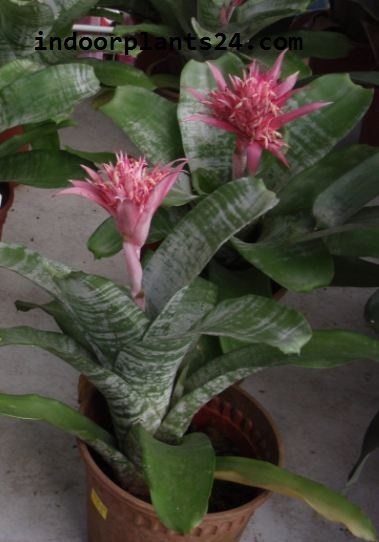The image showcases a detailed view of a succulent plant in a brown pot, situated on a cement or concrete floor. The succulent has thick, waxy leaves with white stripes and features two prominent, intricate, spiky pink flowers that stand out vividly. In the background, which is dark and somewhat indistinct, there are hints of additional plants. The top of the image includes the somewhat difficult-to-read text "IndoorPlants24.com" written in black.